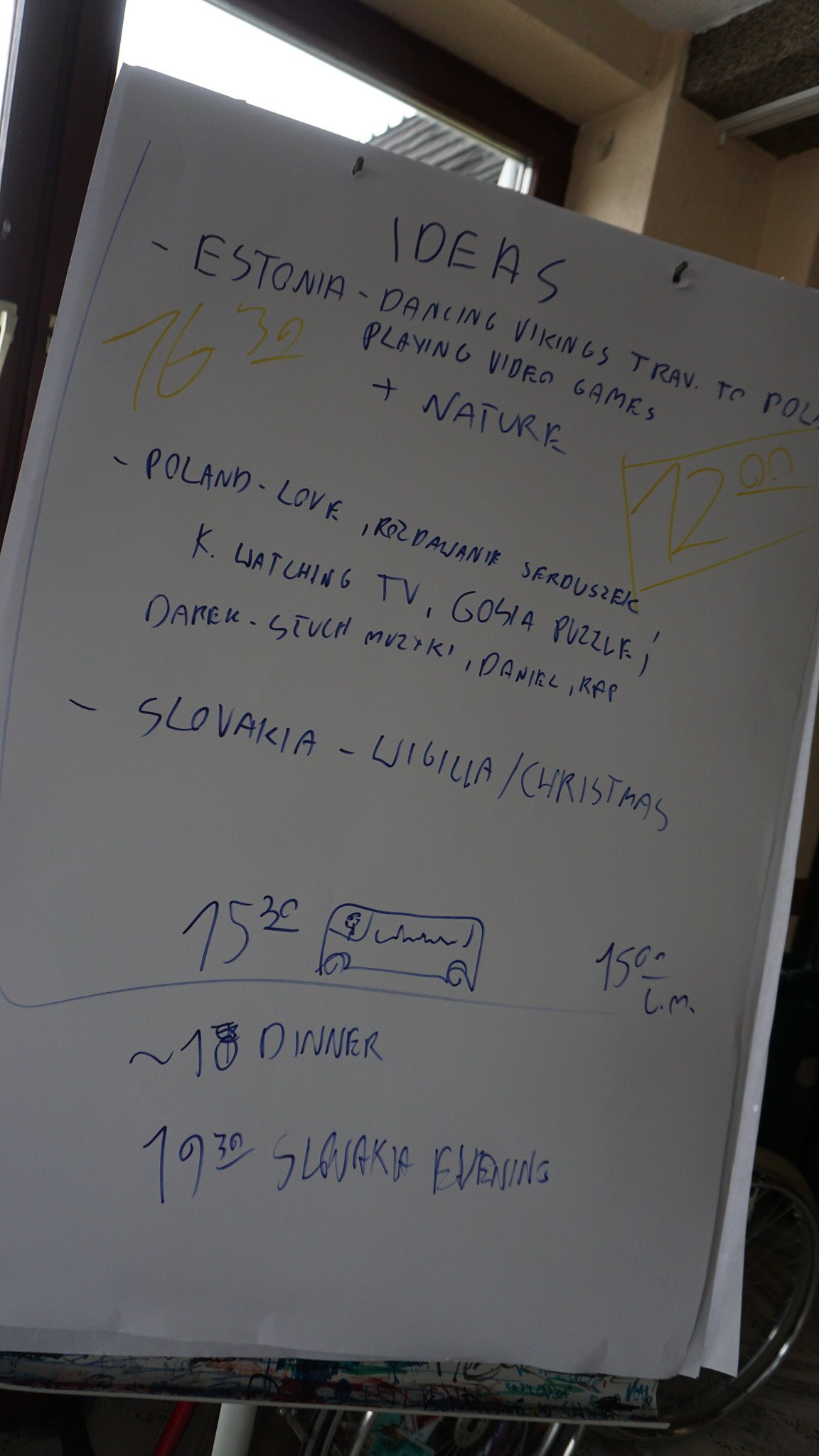This is an up-close photograph of a large white notepad or possibly a dry erase board, filled with handwritten notes in dark blue ink. At the top, under the title "Ideas," the notes are organized with bullet points. The first bullet point lists: "Estonia," followed by "Dancing Vikings," "Train to pole," and "Playing video games plus nature." The second bullet point mentions "Poland," and includes phrases such as "Love Roz," "Darwinian," and "Puzzle," although some words are unclear and not in English. The next bullet point is "Slovakia," followed by "Wigilia/Christmas." 

Below these notes, there's a crude drawing of a bus, with various dollar amounts written nearby: "$75.30," "$76.30," and "$72," the latter encased in a box. There is also a mention of "Dinner" and a time "19:30," indicating possibly a schedule or budget for a trip. The mixture of clear and unclear text, along with the different languages, suggests brainstorming or travel planning.